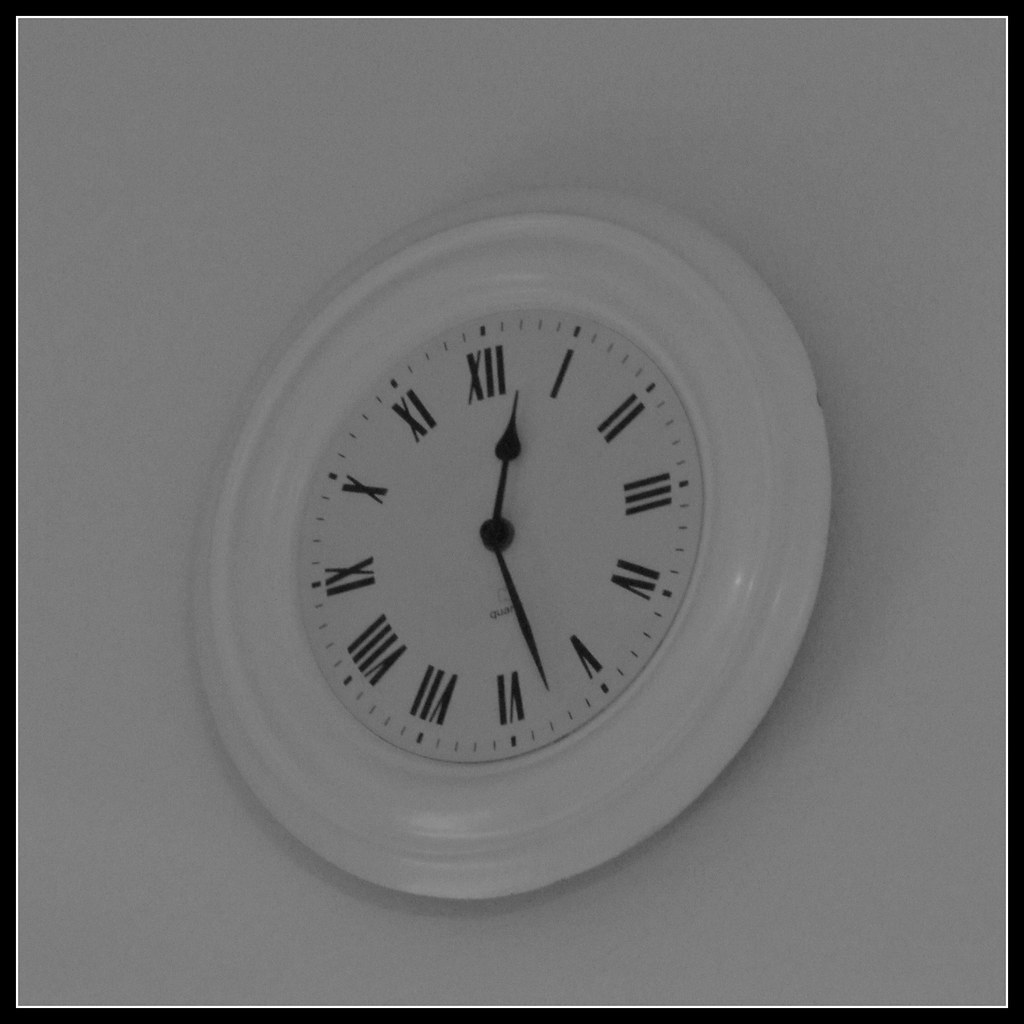This image depicts an extreme close-up of a predominantly smooth wall, which appears to be medium gray due to the lighting. The focal point is a round clock hanging on this wall. The clock features a white face with black Roman numerals arranged from I to XII around its edge. Black tick marks for the minutes are also present, adding to the precision. There are two black hands: the minute hand is narrow and thin, while the hour hand has a slightly ornate arrow pointer. A small text reading "quartz" is located beneath the axle of the hands. This round wooden clock has a ridge along the inside perimeter of its circular frame, and it appears to be positioned slightly off-center towards the 5 o'clock mark, showing a time of 12:27. The clock's border consists of a razor-thin white outline encircled by a slightly thicker black line that contrasts against the wall.